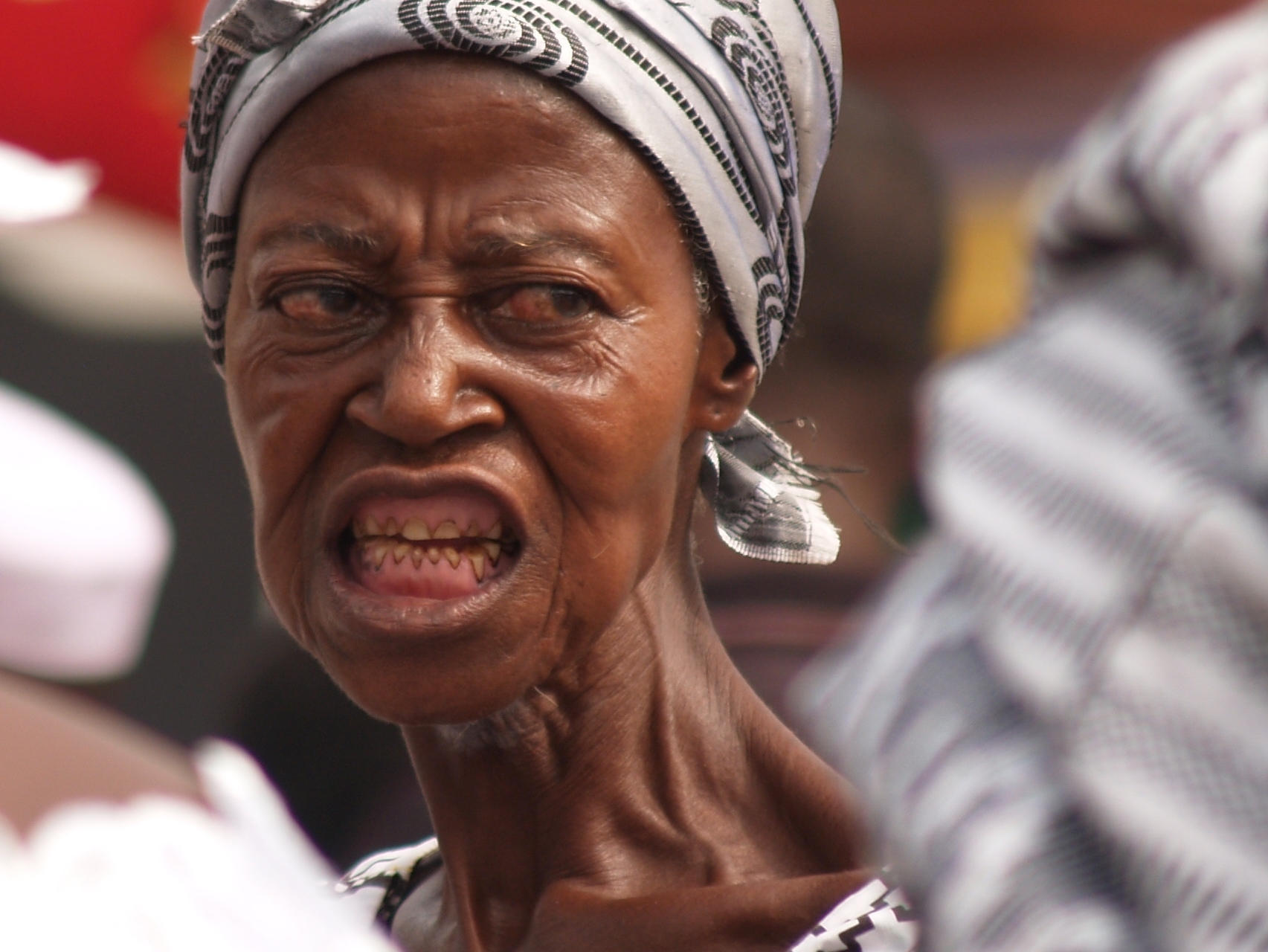In this detailed photo, we see an exceptionally angry Black woman, possibly of African descent, standing outdoors. She has a distinctive headdress tightly wrapped around her head, displaying gray and white swirls, with a small amount of gray hair peeking out near her ears, suggesting she might be older. Her facial expression is striking—her mouth is open wide as if yelling, revealing severely deteriorated gums and abnormally short, discolored teeth, giving an almost unreal or AI-generated appearance. Her eyes are bloodshot with prominent veins and a lack of whiteness, adding to her intense, strained demeanor. She is looking to the left of the image, her neck muscles taut, revealing pronounced collarbones that appear somewhat misaligned. In the blurry background, there is another person wearing a large, striped headdress, also in gray and white hues, and a man with short hair. The scene is shot during the daytime, with the woman sharply in focus, emphasizing her ferocity and unsettling, almost uncanny presence.